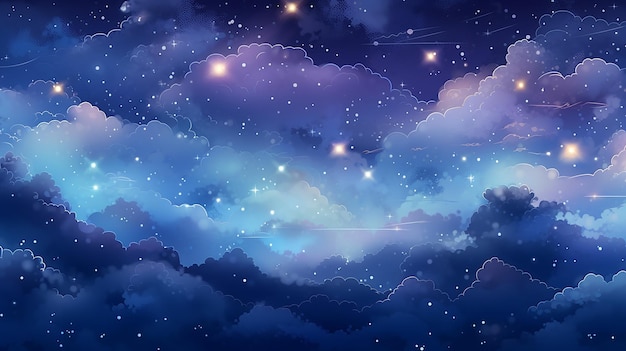The image depicts a beautifully animated night sky, likely from a cartoon or movie, showcasing an array of vibrant colors. The sky transitions from deep blacks and dark purples at the edges to lighter purples and blues toward the center, where the sky becomes a light blue. Dotted throughout this colorful expanse are numerous stars, varying from white to hues of yellow and blue, and larger stars that fade into orange tones. The scene is further enriched with the presence of clouds, some of which appear as faint white outlines, possibly suggesting distant clouds or even shooting stars. These clouds have a distinct scalloped shape, most prominently visible on the right and left sides of the image, while some central clouds appear more transparent. The clarity of the digital painting accentuates the vividness of the colors and the twinkle of the stars, creating a captivating and clear portrayal of a fictional night sky.